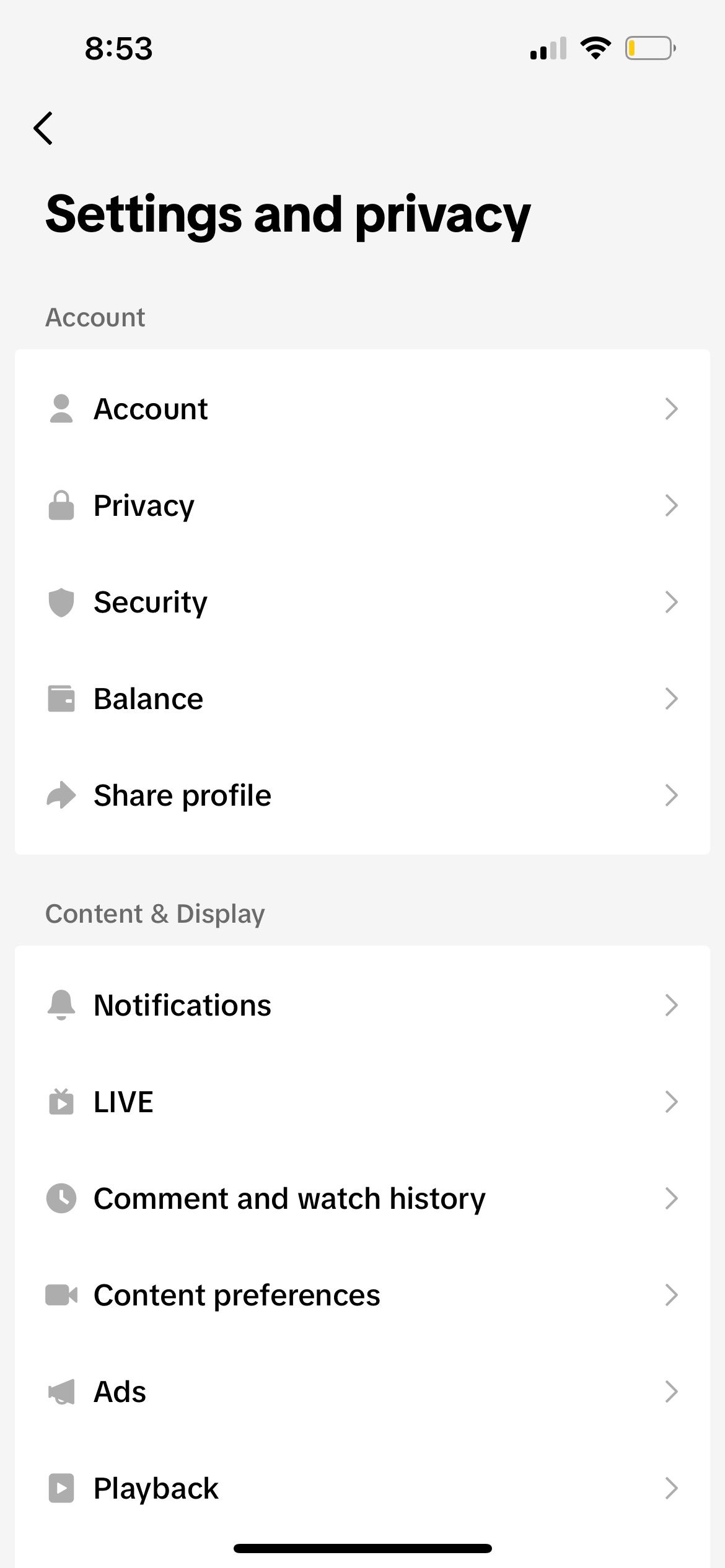A smartphone screen displaying the settings and privacy menu of an application, likely on an Android device given the interface design. The top of the menu is labeled "Settings and Privacy," followed by sub-sections in a list format: Account, Privacy, Security, Balance, Share Profile, Notifications, Live, Comment and Watch History, Content Preferences, Ads, and Playback. Each of these sections features an arrow indicating the presence of further options. The user interface includes a progress bar at the bottom, suggesting the possibility of closing the menu. This appears to be the settings and privacy section of a social media or video application, possibly Instagram or YouTube, though the exact app is not specified.